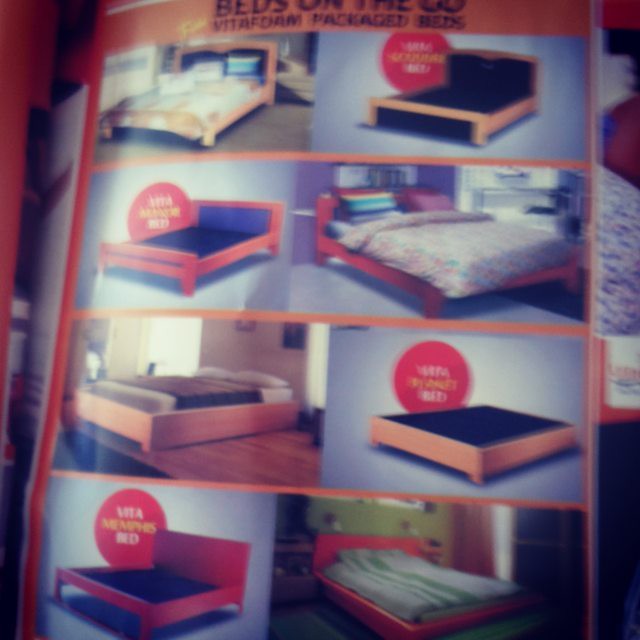This image appears to be an advertisement for bed frames featured inside a magazine. The page is organized into eight panels, each showcasing a different type of wooden bed frame. The frames vary in shades from light to dark wood and are low profile, standing close to the ground on four legs. Each bed in the panels either features a plain black cloth-covered mattress or is neatly made with bedding, ranging from floral patterned sheets to dark solid covers. A distinctive orange outline frames each panel, and at the top of the page, there is partially visible text that seems to read "Beds on the go," followed by "packaged beds," albeit blurry. Red circular stickers are present on four of the bed images, likely advertising deals, though the writing is unclear. The layout alternates, with made-up beds and bare frames with red informational circles placed interchangeably across the rows. The overall appearance is somewhat blurred, making finer details difficult to discern.